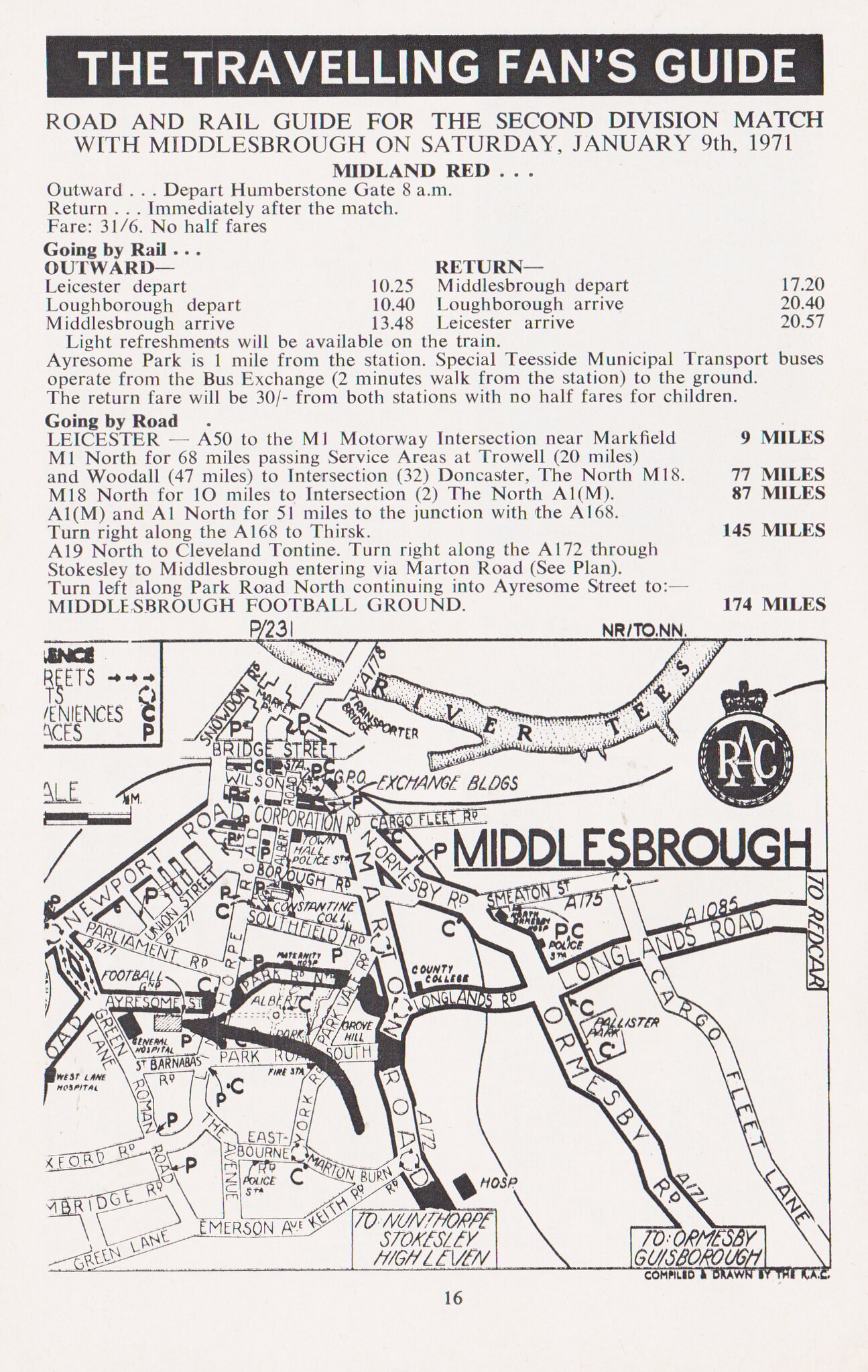This detailed image is a vintage page from a travel guide booklet titled "The Traveling Fans Guide" for the second division match with Middlesbrough on Saturday, January 9th, 1971. Labeled as page 16, it features a hand-drawn map of Middlesbrough, centered and detailed with roads including Newport Road, Parliament Road, Long Lans Road, Erisum Green, Roman Road, and Martin Road, as well as the River Tees. 

At the top of the page, in a black horizontal strip, the guide's title is prominently displayed, while just below it is the subheading detailing the match date. The text provides comprehensive travel information for fans, outlining times and fares for both road and rail transport. 

Rail information includes departures from Leicester at 10:25 AM and Loughborough at 10:40 AM, arriving in Middlesbrough at 1:48 PM. The return journey departs Middlesbrough at 5:20 PM, arriving back in Leicester at 8:57 PM, with light refreshments available on the train. 

For road travelers, the guide details the route via the MI motorway, specifying intersections, service areas, and mileages, ultimately directing fans to Middlesbrough Football Ground via Martin Road. The guide notes that buses from the bus exchange, a two-minute walk from the station, also operate to Erisum Park, which is one mile from the train station. Fares are specified, pointing out there are no half fares for children.

The map is marked with various labels and symbols, including a logo resembling a queen’s crown in a circle at the top right, reading "R A C". The page also includes seemingly incomplete texts in several sections, possibly indicating additional notes or annotations. A footnote at the bottom outside the map border states “compiled and drawn by the RSE.”